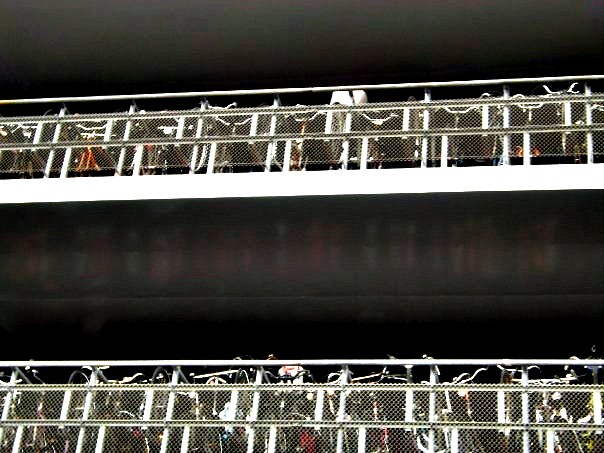The photograph depicts a multi-story bicycle parking garage constructed primarily from concrete, with visible levels showing detailed parking arrangements. The structure reveals at least two floors, each lined with a white chain-link fence that separates individual slots for bicycles. Within each slot, defined by additional white metal bars, numerous bicycles are neatly parked. The bicycles exhibit a range of colors including occasional pops of red and orange, although many are primarily black with chrome details. The lower levels are shaded, adding contrast to the overall gray and white hues of the concrete and fencing. Despite the limited view, there is a noticeable clear pattern of orderly bicycle arrangement within the garage. The setting is devoid of text, emphasizing the stark and functional design of the bicycle storage area.